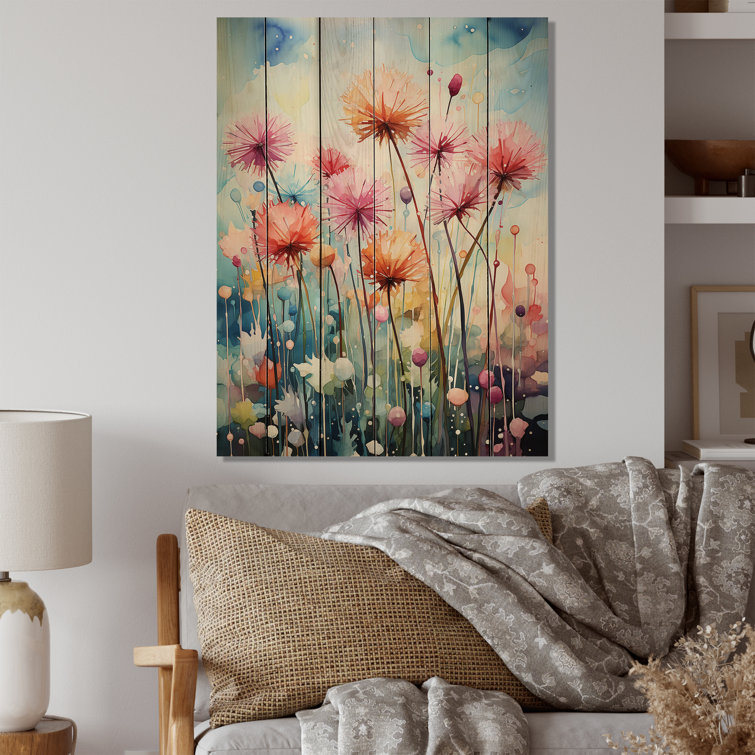This indoor image captures a cozy corner of a living room, showcasing a light tan wooden-framed couch adorned with neutral gray and tan cushions, and a gray throw blanket with a white pattern. The couch sits against a pristine white wall, which prominently features an unframed painting of vibrantly colored dandelions in pink, orange, and yellow hues, executed in watercolor on six wooden planks. The splashes of blue, white, pink, and gray add depth to the visually stunning artwork. To the right of the couch, a white lamp with a matching shade sits atop a wooden nightstand. The background includes built-in shelves displaying a bowl, a framed piece of art, and a book, adding to the room's thoughtful and tranquil decor. A small tan plant peeks from the bottom right, completing this serene living space.